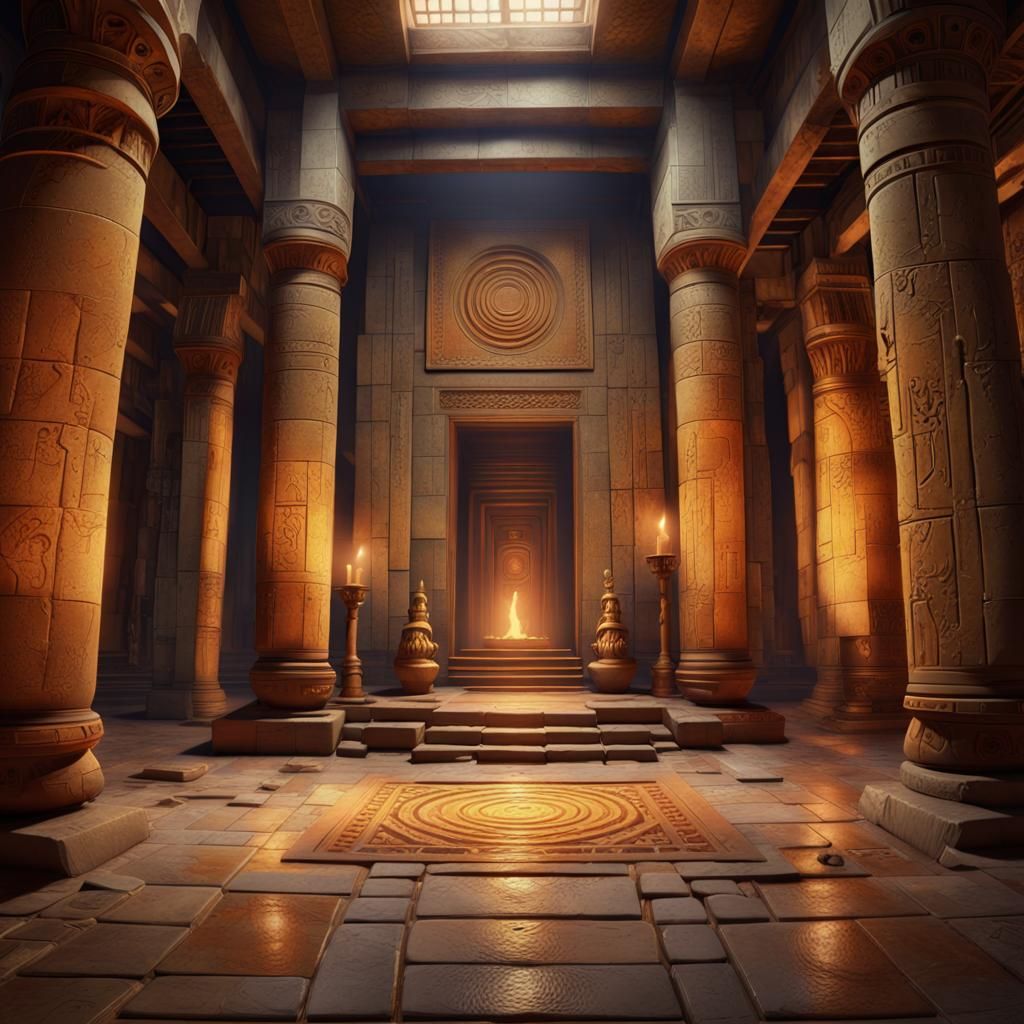The image appears to be an AI-generated depiction of an ancient temple or palace interior, possibly Egyptian. The scene features numerous pillars adorned with intricate designs, arranged in two main rows, creating a grand aisle leading to a raised platform. The floor is composed of large stone slabs, with a gold inlay forming a circular pattern in the center of the aisle. Flanking the steps that lead up to the platform are two large, ornate vases. At the top of the steps, we see a significant fire pit with a high flame, adding a dramatic focal point. Additionally, candles or fire sticks are placed on some of the pillars near the steps. The high ceiling and overall grandiose architecture of the space give the impression of a significant ceremonial hall or a sacred temple chamber. There is no text within the image to provide further context.